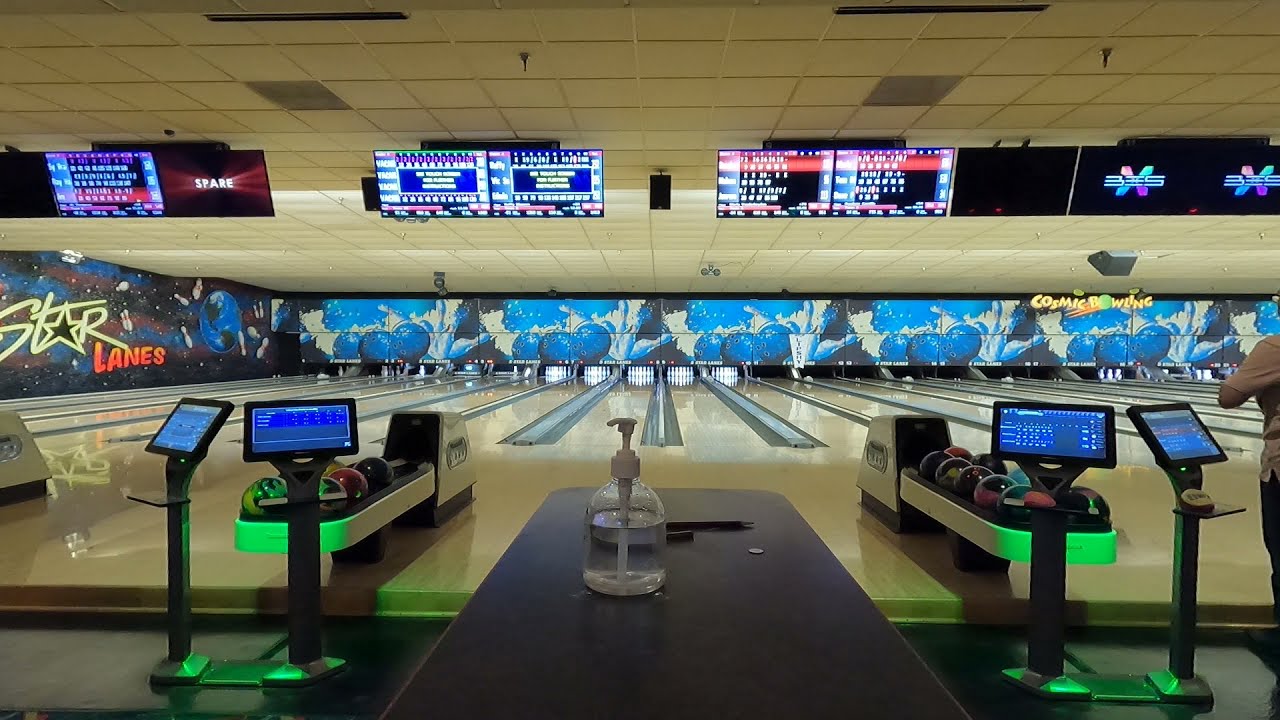The image captures a modern bowling alley called Star Lanes. The vantage point is from behind a thin desk or table positioned between two lanes, adorned with a bottle of hand sanitizer and a pen. The expansive view ahead reveals about 15 lanes, each equipped with colorful bowling balls and digital score monitors. The lanes themselves are a creamy white color, converging into a sleek black bowling floor where the ball returns are situated. Hanging from the ceiling are multiple digital displays showing scores, with one screen prominently displaying the word "Spare" in bright white letters against a red background. In the background, there are banners and murals: one with three large blue bowling balls appearing to erupt into pins amidst blue and white smoke, and another showcasing the Star Lanes logo against a constellation-themed backdrop with Earth and floating pins. A single person in a white shirt and black pants is partially visible on the right side of the image, adding a hint of human activity to the otherwise serene scene. The ceiling is composed of a typical square drywall board, completing the crisp, modern aesthetic of the bowling alley.